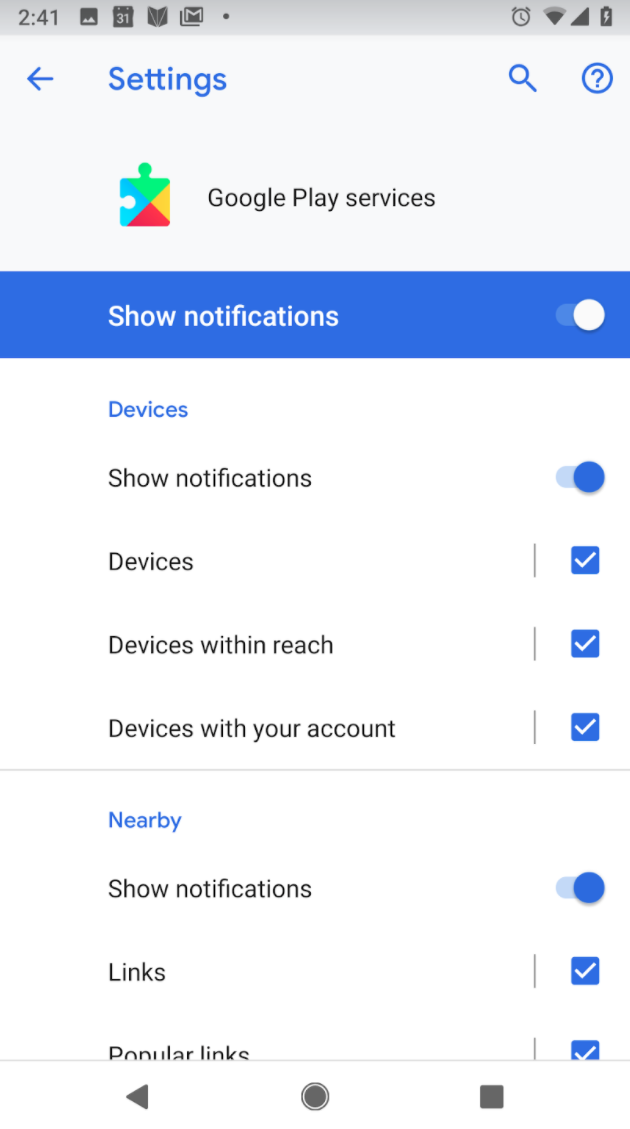Here's a cleaned-up and detailed descriptive caption for the image:

---

This mobile screenshot captures the settings tab in Google Play. At the top left, the word "Settings" is displayed with a left-pointing arrow beside it. In the top right corner, there are icons for a magnifying glass and a question mark. Below these icons, centered on the screen, are the words "Google Play services" written in black text, accompanied by a multicolored puzzle piece icon representing Google.

Directly beneath this section, a blue banner with white text reads "Show notifications," and to the right of this banner is a toggle switch that is currently turned on. The background below is predominantly white, featuring various categories and their settings.

The first category titled "Devices" is highlighted in blue. Under this category, "Show notifications" appears again with a corresponding toggle switch that is also turned on. The word "Devices" is followed by a checkbox, which is checked. Two more options under this category, "Devices within reach" and "Devices with your account," each have checkboxes that are checked as well.

The next category listed is "Nearby," also highlighted in blue. Under this section, "Show notifications" once more includes an enabled toggle switch. The options "Links" and "Popular links" are indicated as clicked. 

The remainder of the screenshot would require scrolling down to view additional settings.

---

This detailed caption provides a comprehensive description of the entire visible content in the screenshot.